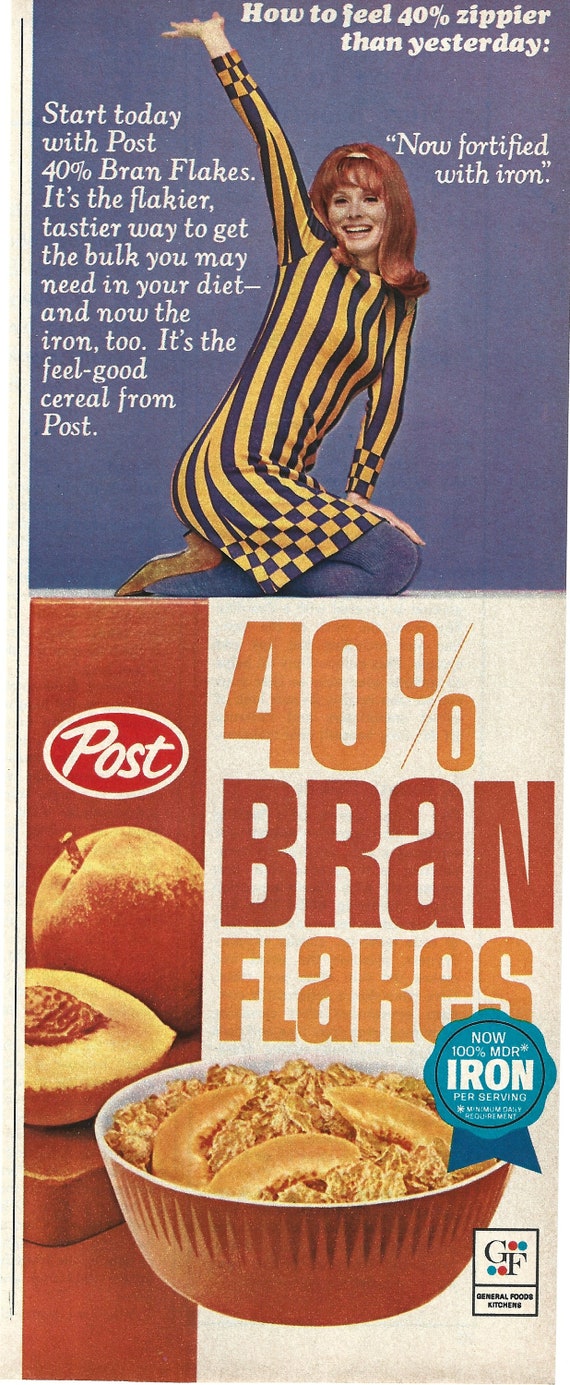The image appears to be a vintage advertisement, split into sections against a blue background. Dominating the upper section, white text reads, "How to feel 40% zippier than yesterday. Start today with Post 40% Bran Flakes. It's the flakier, tastier way to get the bulk you may need in your diet—and now the iron too." Below the text stands a woman with long, puffy brown hair that curls around her shoulders, dressed in a striped yellow and blue mini dress paired with blue leggings and brown high heels. She is depicted smiling, throwing her right arm into the air while her left hand rests on her lap. Intriguingly, she appears tiny, as if she's standing atop a large cereal box, indicating humorous scale. The cereal box, prominently below her, features a vibrant red bowl filled with bran flakes and fruit slices, accompanied by the bold text, "40% Bran Flakes" and "Now 100% Fortified with Iron." The Post logo is also visible, pulling the classic advertisement together with a nostalgic touch.